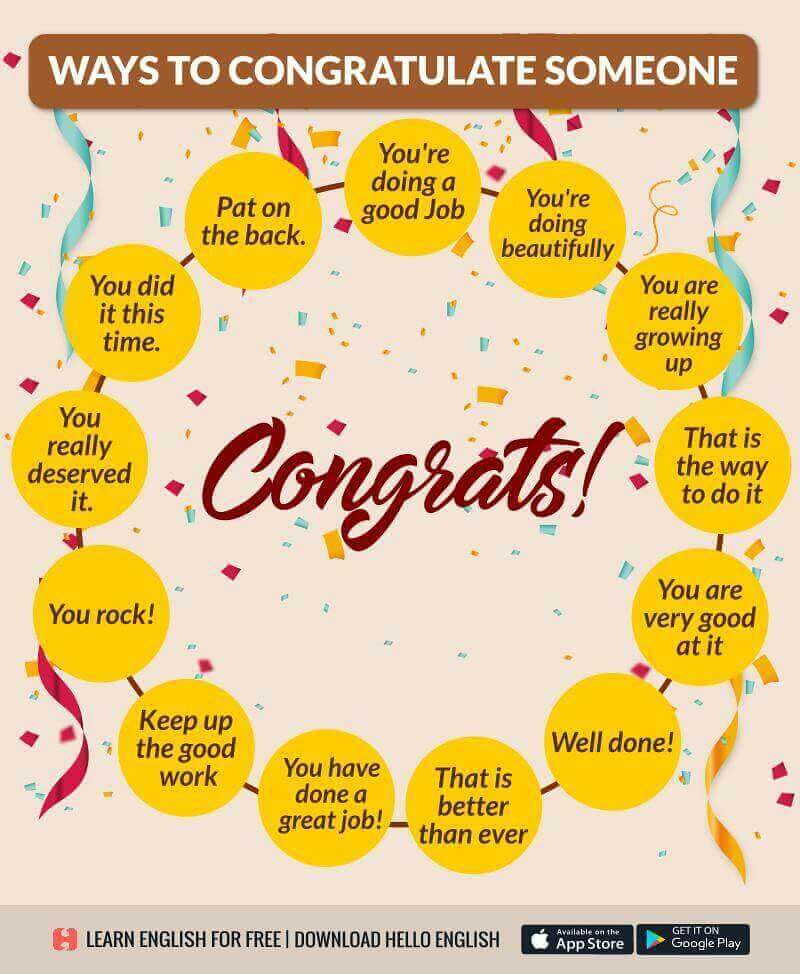The image features a display graphic with a grayish-pink background that might be from a website or printed pamphlet. At the top, a brown rectangular bar with white text reads, "Ways to Congratulate Someone." Surrounding the center, yellow circles form a larger circle, each linked by brown lines. Inside these circles, written in brown font, are various congratulatory messages including, "You're doing a good job," "You're doing beautifully," "You are really growing up," "That is the way to do it," "You are very good at it," "Well done," "That is better than ever," "You have done a great job," "Keep up the good work," "You rock," "You really deserved it," "You did it this time," and "Pat on the back."

In the center of the circle, the word "Congrats!" is written in crimson red cursive, surrounded by flying confetti in red, blue, and yellow. At the bottom of the image, on a light gray bar with dark lettering, a promotional message reads, "Learn English for Free. Download Hello English," accompanied by icons for the App Store and Google Play.